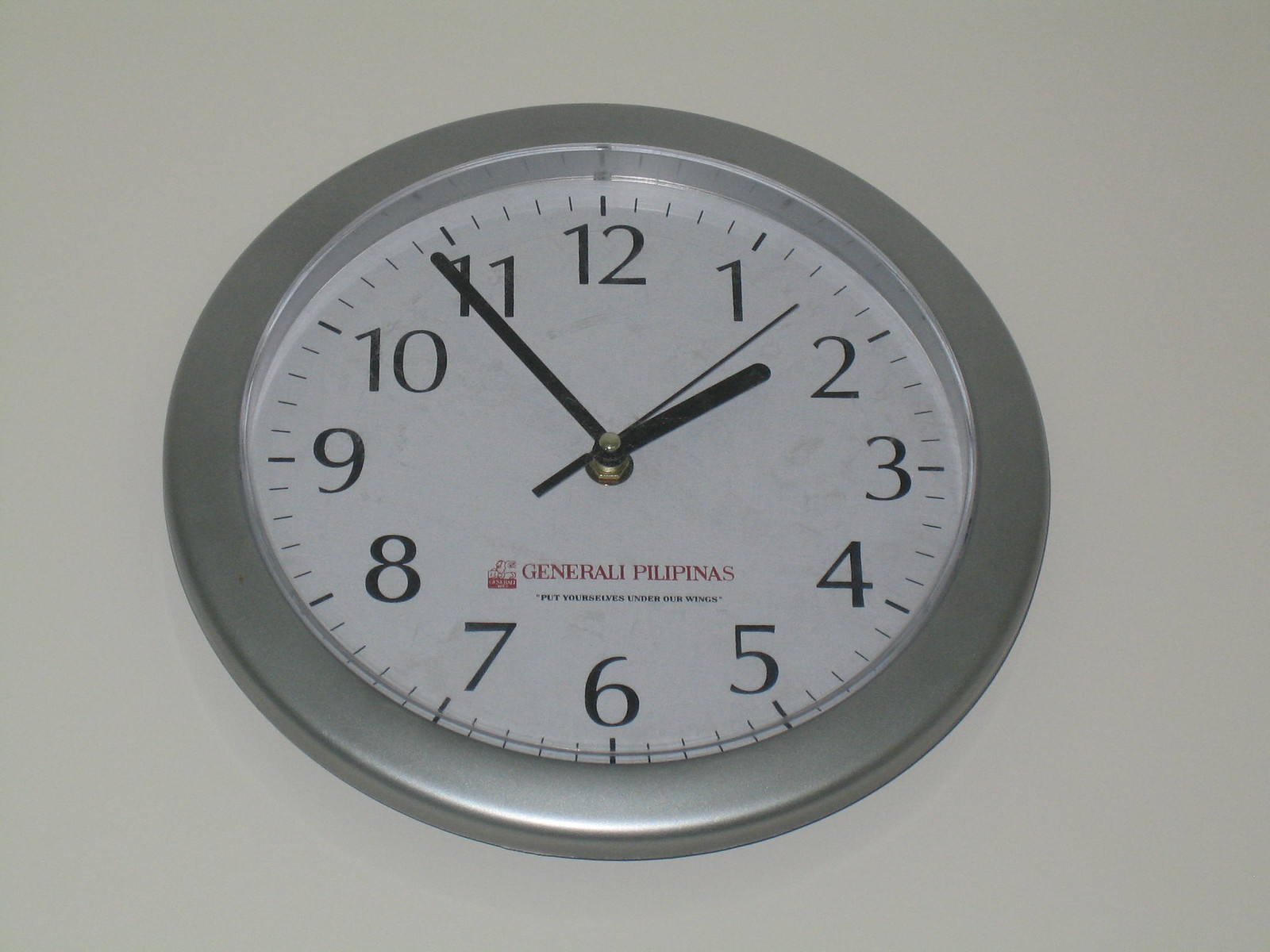In this photo, there's a clock mounted on a grayish-white wall, indicating an office setting. The clock is perfectly circular with a thick gray trim surrounding it. It features a clear plastic cover, a white background, and black font for the numbers and all the smaller notations between the hours. The current time displayed is approximately 1:55. The numerals are in a bold black font, as are the hour, minute, and second hands. Near the bottom of the clock face, the text "GENERALI PILIPINAS" is prominently displayed in all capital letters in red. Adjacent to this text is a red logo, and beneath it, there is some additional text that is not clearly visible in the photo.